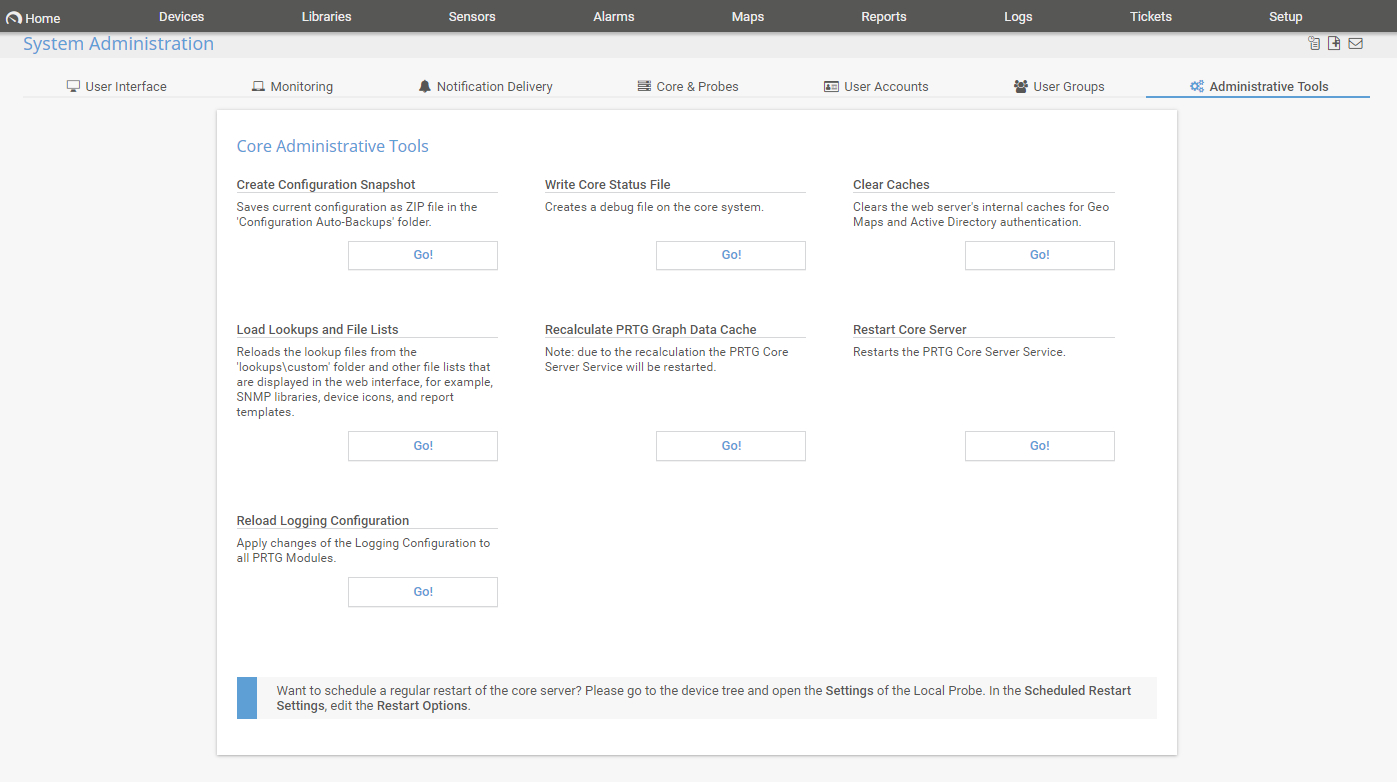The interface display showcases a black navigation bar at the top, offering a series of clickable options from left to right: Home, Devices, Libraries, Sensors, Alarm, Maps, Reports, Logs, Tickets, and Setup. Beneath this, on the left side, the text "System Administration" is emphasized in blue, accompanied by several indistinguishable icons. On the right side of this header arrangement, an image is displayed. Below the header, a secondary navigation line lists further clickable options: User Interface, Monitoring, Notification Delivery, Core and Probes, User Accounts, User Groups, and Administrative Tools. Underneath this segmented menu, a white box labeled "Core Administrative Tools" details specific functions, such as Create Configuration Snapshot, Write Core Status File, Clear Cache, Lookup and File Lists, and Restart Core Server. This intricate interface appears designed for comprehensive system management and administrative tasks.